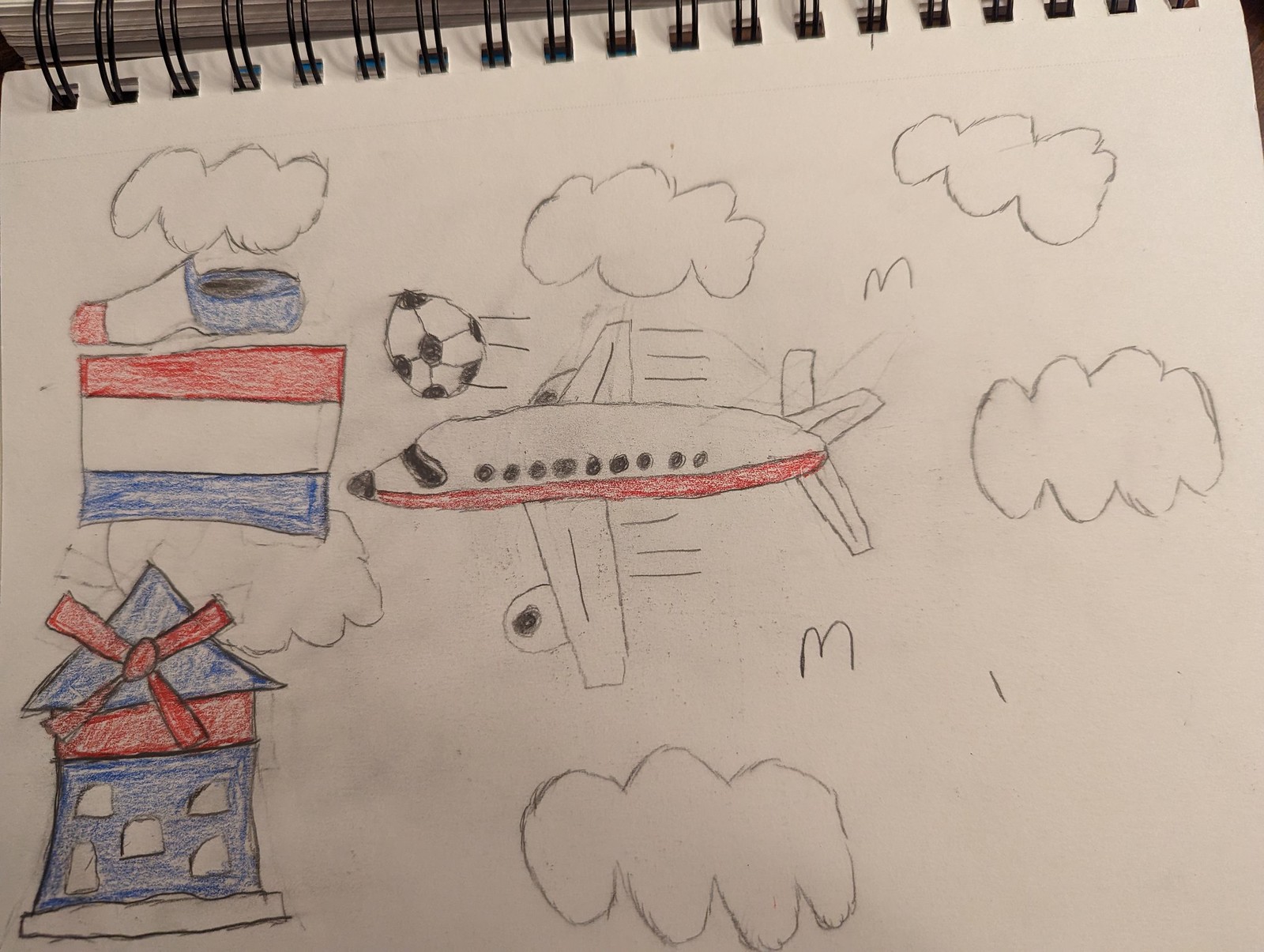This image is a photograph of a child's drawing, depicting a lively and imaginative scene. At the center of the drawing is a jet airplane with a sleek, white body, a red stripe running along its side, and a black nose. The plane is soaring through the sky, surrounded by fluffy clouds. In an interesting twist, a soccer ball is drawn above the airplane, streaking through the sky with motion lines, suggesting it is flying. The airplane's nose is pointed towards a flag striped with red at the top, white in the middle, and blue at the bottom. Above this flag, there is an intriguing depiction of a wooden clog, decorated similarly with a red tip, white midsection, and blue heel. In the bottom left corner of the drawing, there is a charming red, white, and blue windmill, adding a whimsical touch to the entire scene.